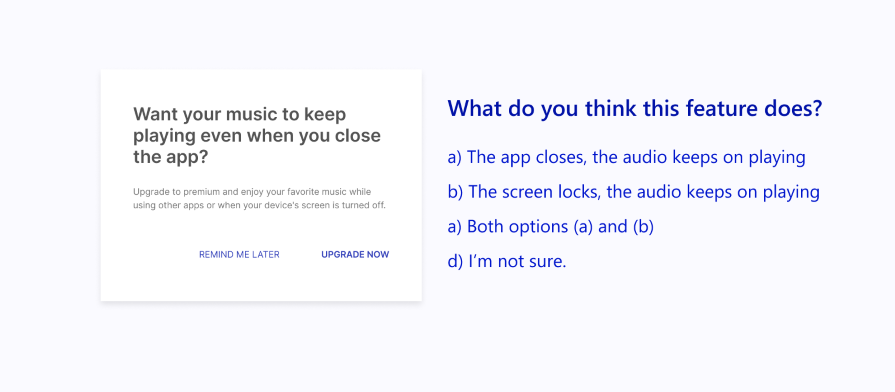The image features a clean and minimalistic interface with a lilac pink or lilac purple background. At the center, there's a prominent white box with text that reads, "Want your music to keep playing even when you close the app? Upgrade to premium and enjoy your favorite music while using other apps or when your device's screen is turned off." Below this text are two clickable buttons: one labeled "Remind Me Later" and the other "Upgrade Now."

To the right of the white box, a question appears in blue text: "What do you think this feature does?" The multiple-choice options are listed as follows:
- A: The app closes, the audio keeps on playing.
- B: The screen locks, the audio keeps on playing.
- A: Both options A and B.
- D: I'm not sure.

There is a notable error in the labeling of the options, with two options labeled as "A" instead of the expected sequence of A, B, C, D.

The white box and its contents resemble prompts commonly seen in services like YouTube Premium, which offer features allowing continuous audio playback even when the screen is off.